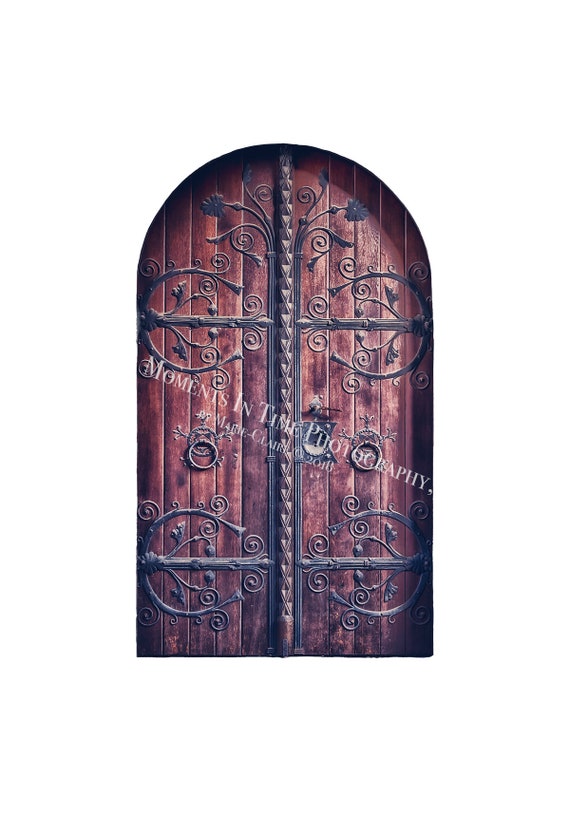The photograph depicts a grand, arch-shaped wooden door reminiscent of those seen in medieval times. The door is central to the image, framed with intricate metal overlays in patterns and designs, including arrows, flower shapes, and curves, in shades of gold, black, and gray. The door, which is set against a white background, is sectioned into four parts and features two handles with knocking hooks in the center. A black metal chain dangles down from it. The watermark text, "Moments in Time Photography by Mary Claris 2018," is prominently displayed in white on the door, indicating it is part of a professional photography series. The door's rich brown wood and the contrasting metal decorations make for a striking, detailed visual.